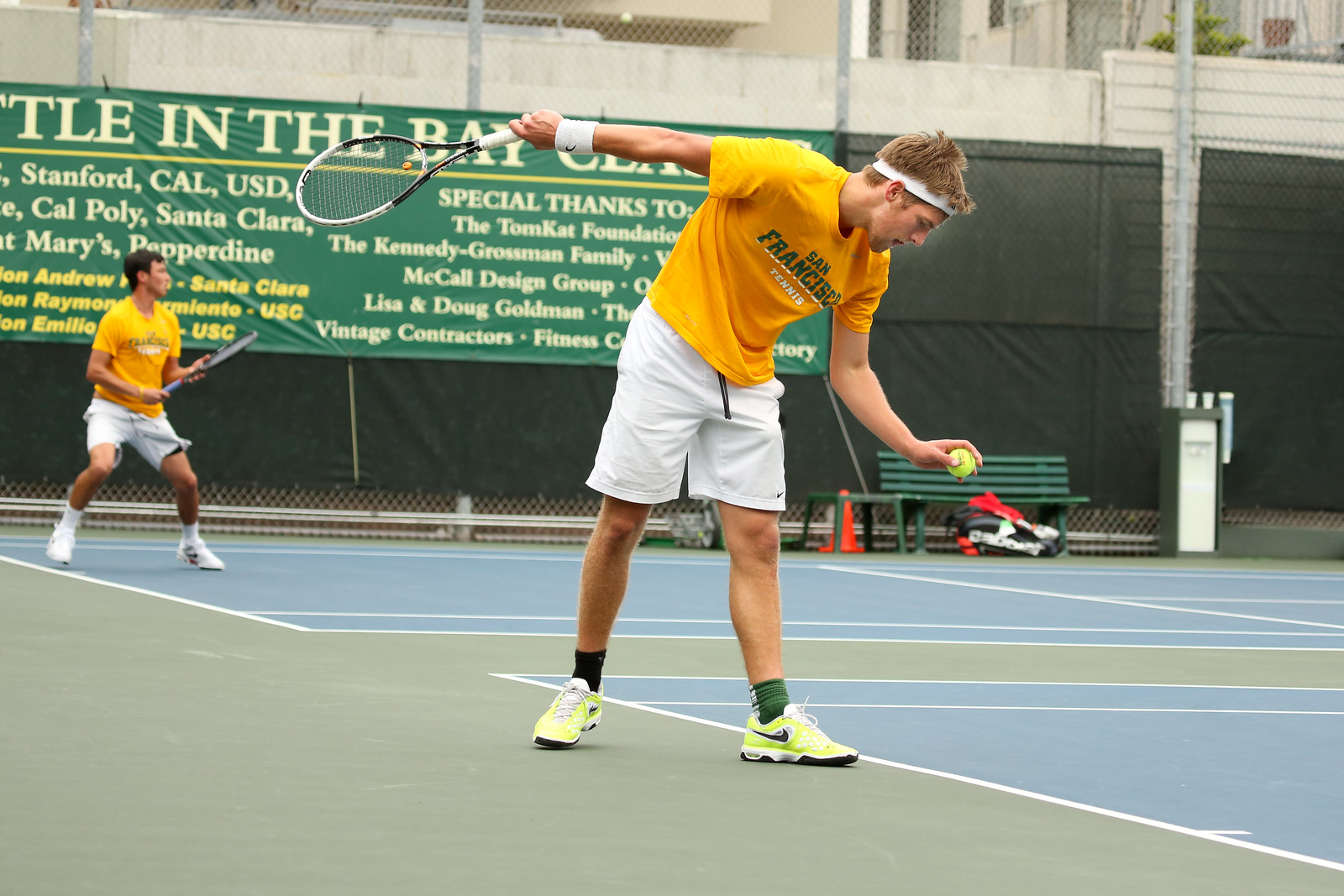The image depicts two men playing tennis on side-by-side courts at a tennis camp or center, indicated by their matching uniforms. Both wear bright yellow shirts with green lettering that reads "San Francisco" and underneath, in white, "tennis." They are also sporting white shorts. The player in the foreground is preparing to serve, with the ball in his left hand and his racket drawn back in his right. He has reddish-blonde short hair, a goatee, and is accessorized with white terrycloth wristbands and headbands. He also wears green socks and yellow Nike tennis shoes. In the background, the second player, in an identical uniform but with white shoes and no headbands or wristbands, appears poised to receive the serve. It's a well-maintained facility, possibly linked to an institution in the Bay Area or a local college.